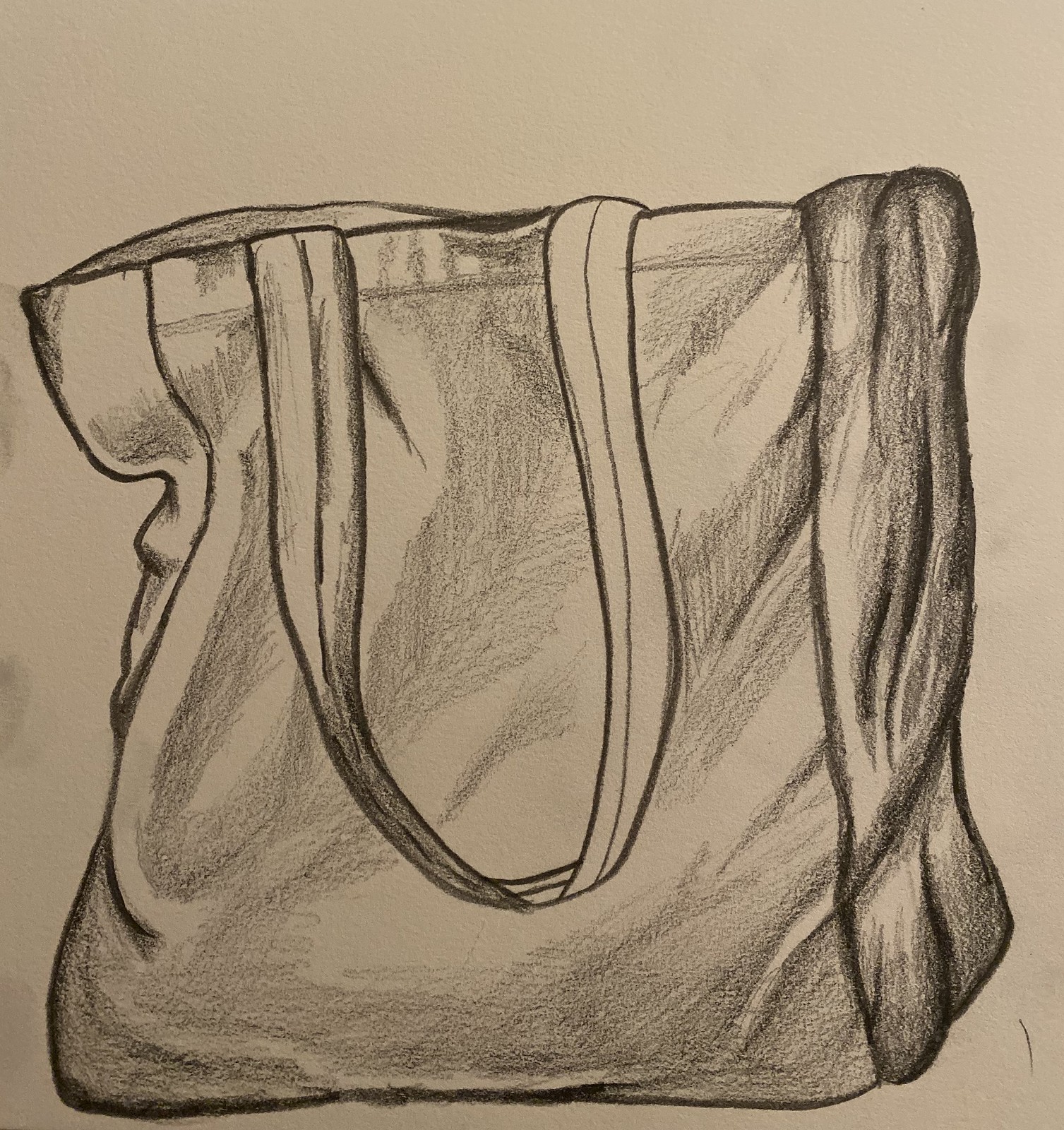A detailed charcoal drawing prominently features a purse against a tan background reminiscent of a grocery store paper bag. The depiction focuses on the left side handle of the purse as viewed by the observer. The handle appears to have fallen over, suggesting the purse is slightly deflated and not filled to capacity. The artist has skillfully utilized shades and shadows to render the bag's structure and dimension, adding a realistic touch to the artwork. The composition is horizontally oriented, showcasing the purse lengthwise rather than from the middle. Overall, the well-executed shadowing and the unique choice of background color enhance the visual appeal of the piece.